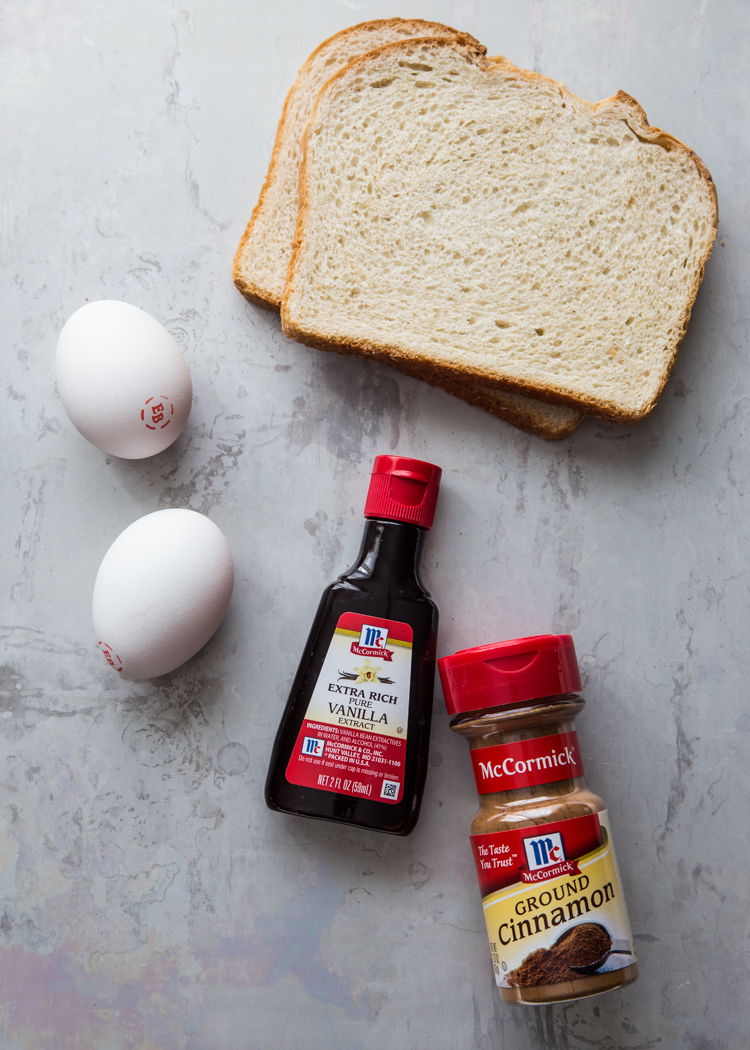This photograph showcases the preparation for making French Toast, with all ingredients neatly arranged on a white marble countertop. There are two slices of white bread laying prominently on the surface, both showing slight dents on the top. To the left of the bread, two eggs, each bearing a red stamp indicating they may be organic or cage-free, are positioned side by side. Centrally placed is a bottle of McCormick Extra Rich Pure Vanilla Extract, signaling the use of authentic flavoring. To its immediate right lies a bottle of McCormick Ground Cinnamon, another essential spice for this breakfast dish. Though there are no additional tools or syrup visible in the frame, it’s clear that the scene is set for someone to whisk the eggs with vanilla and cinnamon, coat the bread slices, and fry them to create delicious French Toast.